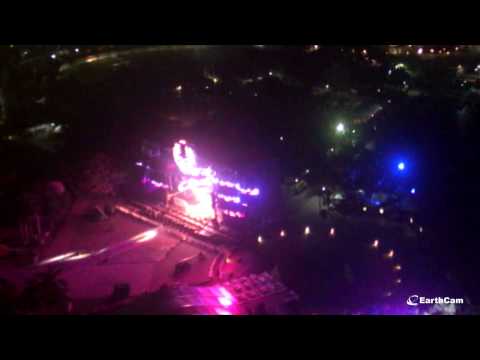This aerial image, likely captured by a surveillance or news camera indicated by the "EARTHCAM" label in white font at the bottom right, presents a nighttime scene. The image's composition is quite dark overall, punctuated by numerous small, scattered points of light, reminiscent of streetlights or house lights. A notable feature is a concentrated area on the left, which is intensely illuminated and possibly indicative of a performance venue with what seems to be a stage or screen. This bright section is surrounded by what appear to be parked cars, suggesting an event or gathering. The lights in this central area exhibit a mix of colors, including light white and reddish hues, while a conspicuous large blue light and a large white light are positioned at an angle on the far right. The top and bottom edges of the image are bordered by black strips, further emphasizing the array of lights, and hinting at the bustling, yet mysterious nighttime activity below.